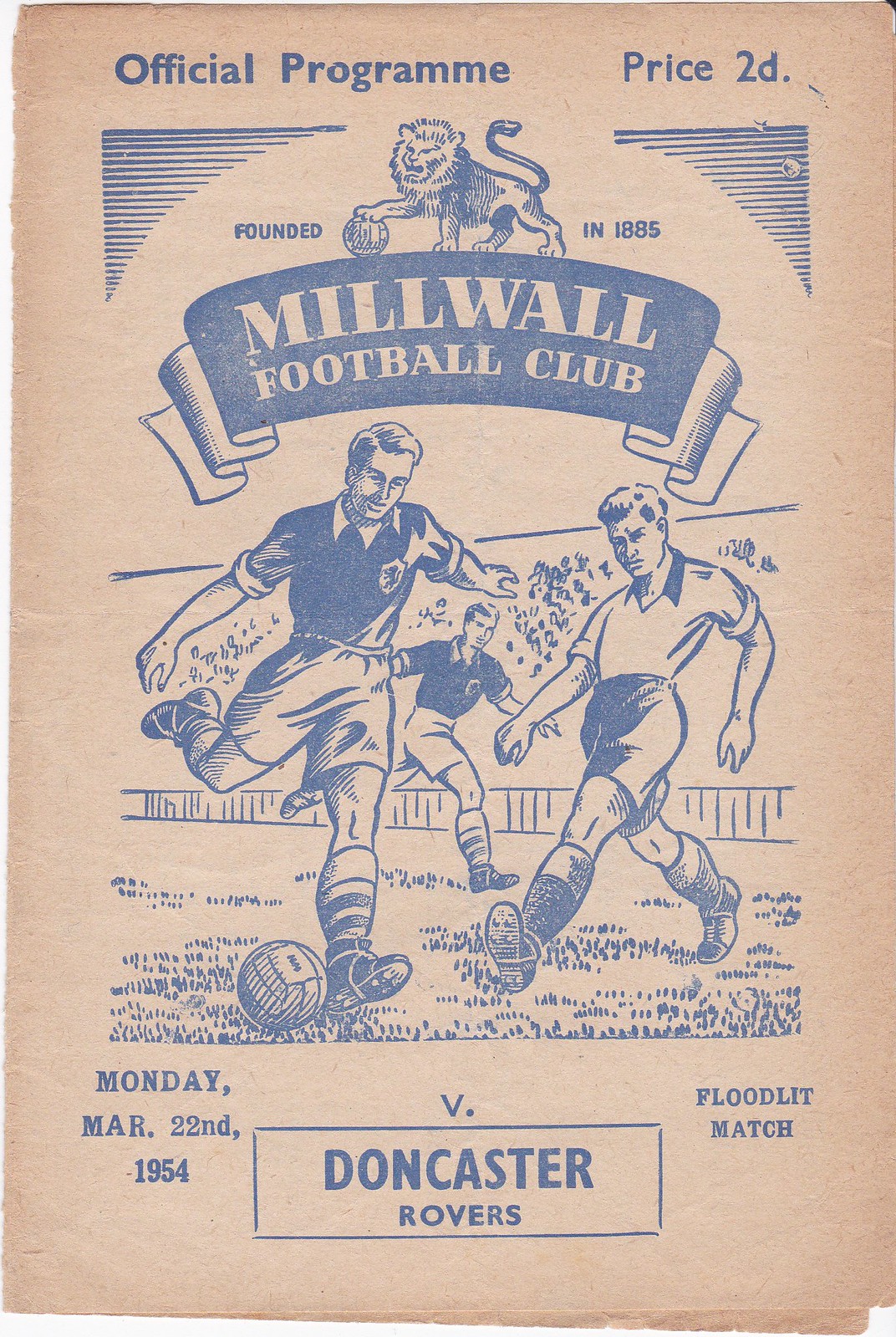This image depicts a vintage Millwall Football Club program dated Monday, March 22, 1954, for a floodlit match against Doncaster Rovers. The background appears to be worn, with a faded beige color, suggesting the original paper might have been white. At the top, "Official Program" is prominently displayed in blue ink, with the price marked as "2D" on the top right. Below, there's a detailed blue illustration of a lion holding a soccer ball, with a ribbon below reading "Millwall Football Club." The centerpiece of the program features a drawing of three soccer players on a pitch, two in darker uniforms and one in a lighter uniform, with one player kicking the ball. Hints of grass and stadium stands are visible in the background. At the bottom, also in blue, it states the match details: "Monday, March 22, 1954, Millwall vs. Doncaster Rovers" and "Floodlit Match."